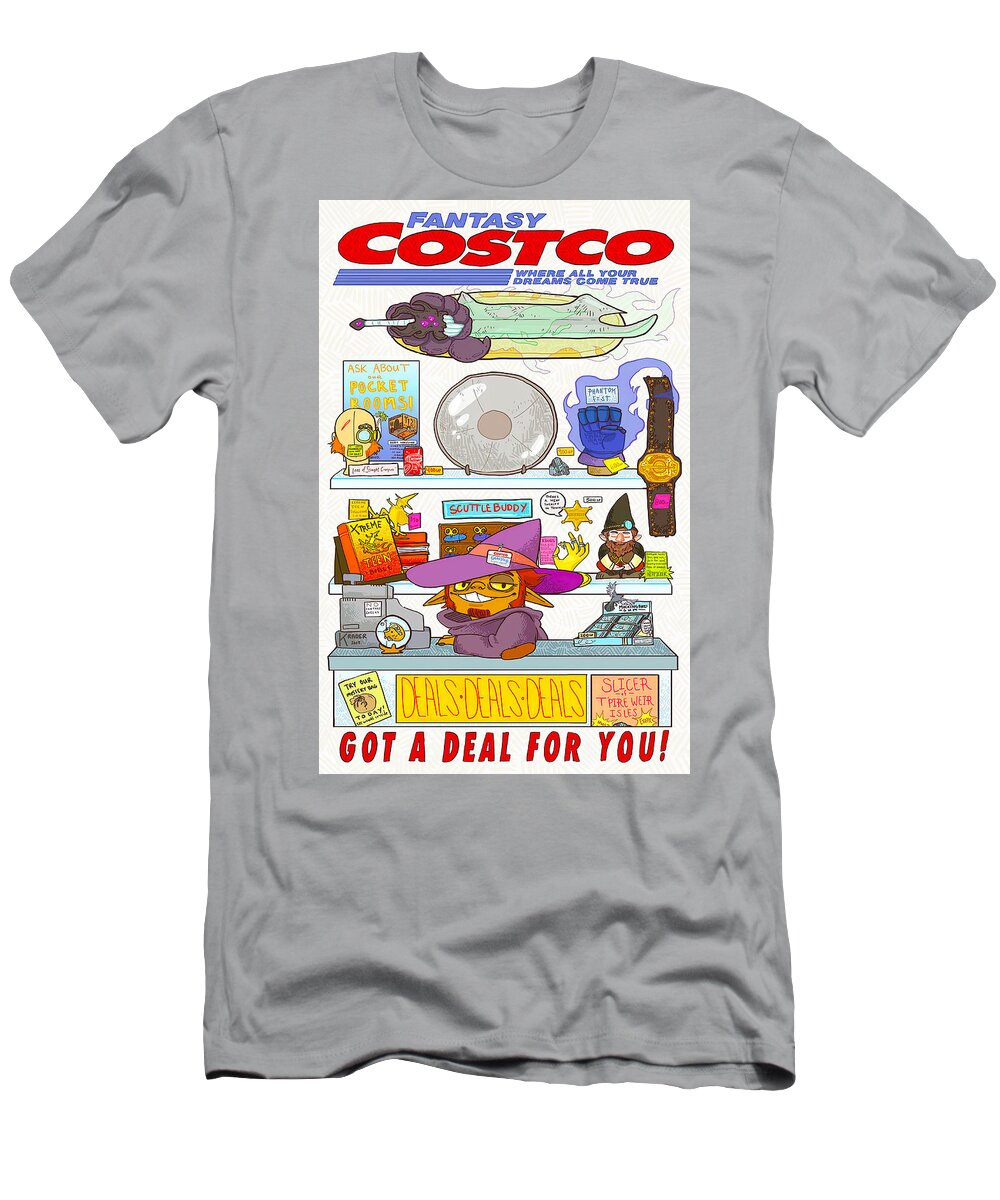The image is of a gray short-sleeve t-shirt featuring a vibrant, whimsical design labelled "Fantasy Costco, where all your dreams come true." The shirt showcases a spoof store layout with a variety of fantasy-themed items. At the top, there appears to be a smoking joint, and below it, a myriad of intriguing objects such as a book, a plate, and a blue fist adorned with a wristwatch. Further down, the design includes another red book, a product called "Scuttle Buddy," and a gnome with a sheriff's badge. The bottom row features a cash register beside a cat-like character wearing a purplish-pink witch's hat, seemingly acting as the shopkeeper. This feline figure is poised behind the counter, exuding eagerness to make a deal, next to a sign that enthusiastically proclaims "Deals, deals, deals, got a deal for you." The background includes shelves laden with playful items like toy swords, comic books, and Dungeons and Dragons tchotchkes, creating a nostalgic nod to 90s gaming culture. The design is set within a white frame on the shirt, rendering an inviting and fantastical shopping scene.